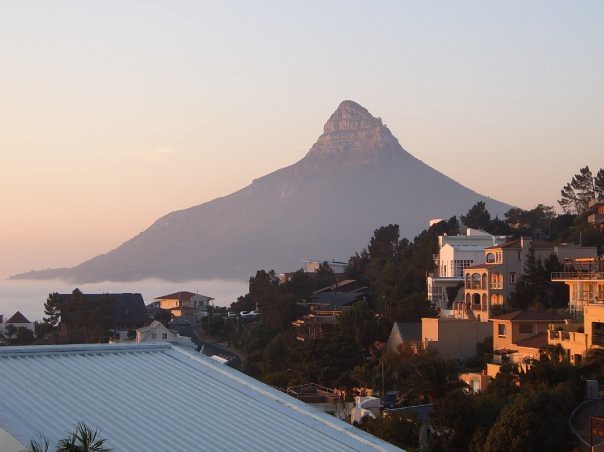This outdoor scene captures a breathtaking landscape dominated by a tall, rocky mountain or possibly a volcano, silhouetted against a sky that transitions from light blue to an orangish-red hue near the horizon. Encircled by water, the mountain rises prominently, its peak barren of any foliage. The image's foreground on the left features a blue, likely tin, roof of a building, hinting at a town setting. Scattered homes, nestled among abundant leafy green trees, dominate the middle ground. The serene beauty of the area is highlighted by the interplay of natural elements—lush greenery, expansive water, and the imposing mountain—all contributing to the image’s tranquil and picturesque atmosphere.